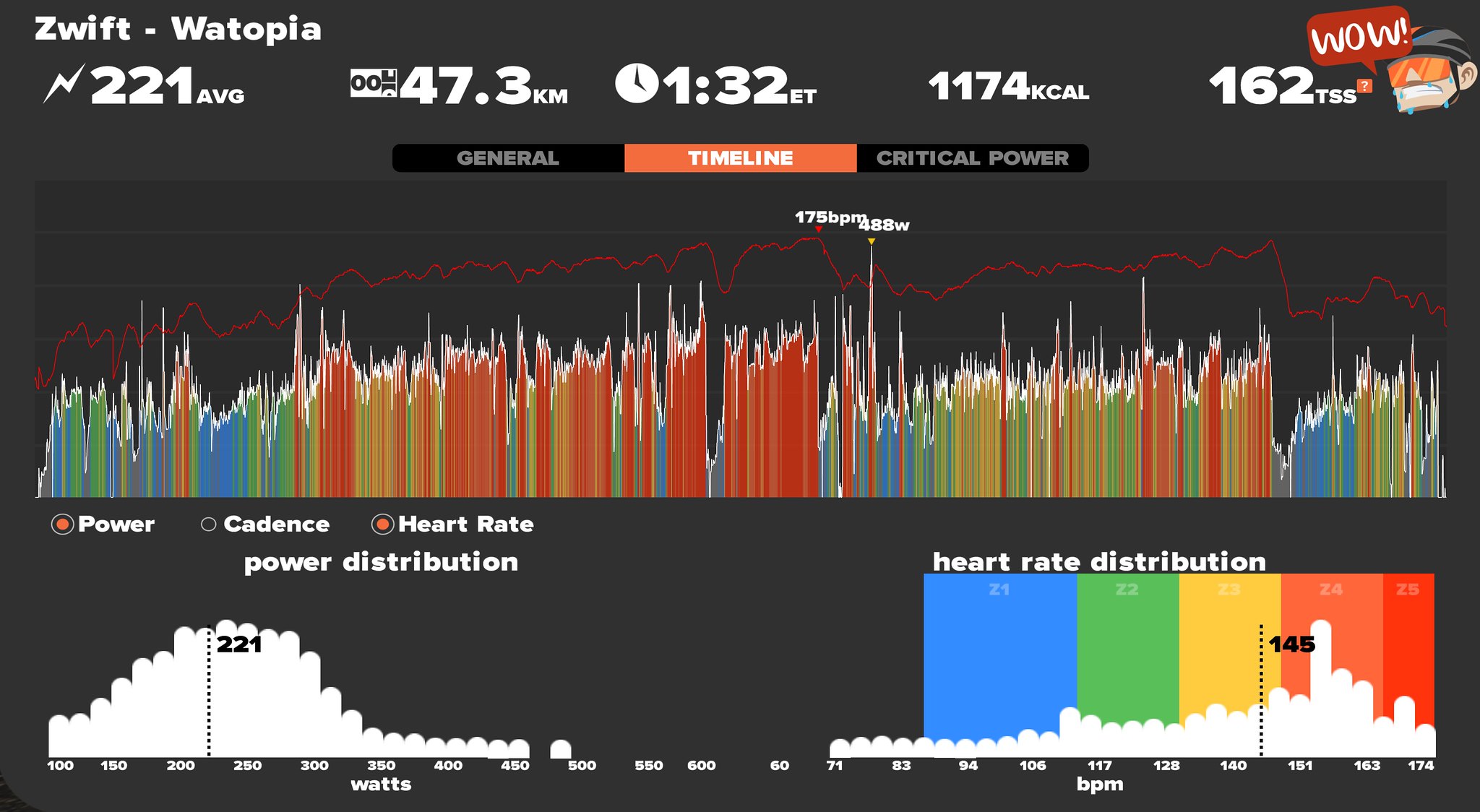The image displays a detailed dashboard of fitness metrics titled "Zwift Watopia" at the top, in white letters. Beneath this title, a lightning bolt icon is accompanied by the figure "221 average," followed by the distance "47.3 kilometers." Further right, a clock icon shows "1:32 ET." Adjacent figures indicate "1174 kilocalories" and "162 TSS." Below this header, a menu bar offers three options: "general," "timeline," and "critical power," with "timeline" highlighted in orange and the others in black. 

Directly underneath the menu bar, the main graph exhibits fluctuating patterns resembling a heart rate monitor, using blue, green, orange, and yellow lines. Below this graph, a section labeled "power distribution" appears on the left, while "heart rate distribution" occupies the lower right corner. These sections feature bar graphs in diverse colors - blue, green, yellow, orange, and red - representing various data points, including power, cadence, and beats per minute (BPM). The entire setup rests on a black background, making the colorful elements stand out.